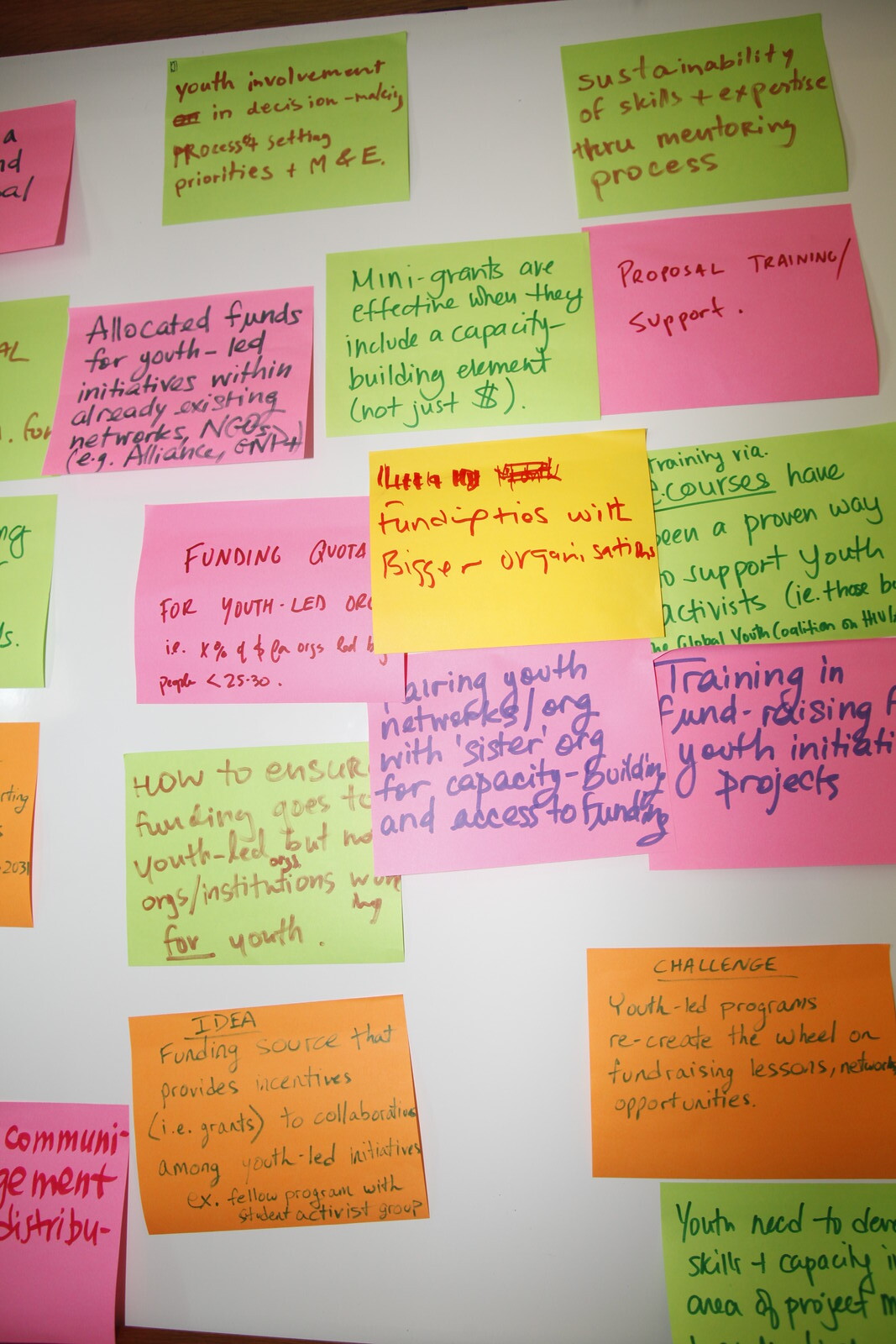The image depicts a whiteboard or possibly a white poster board covered with over a dozen multicolored sticky notes, primarily in shades of light green, yellow, pink, and orange. The scene is a likely result of a brainstorming session, with the focus tightly on the sticky notes, some of which are cropped out on the left and right edges. Each sticky note is inscribed with handwritten text in various ink colors, predominantly red, dark green, and purple, suggesting contributions from different individuals. Notable messages include "youth involvement in decision-making process setting priorities" on a green note in red ink near the top center, "sustainability of skills plus expertise through mentoring process" at the top right, and various other notes discussing topics like "allocated funds for youth-led initiatives" and "many grants are effective when they include a capacity building element." The white background dominates the image, with a partially visible wall in the top and bottom left, possibly in brown or black, adding a marginal contextual detail. This collage of sticky notes encapsulates a collaborative effort, touching upon themes of youth involvement, funding, mentoring, and organizational strategies.